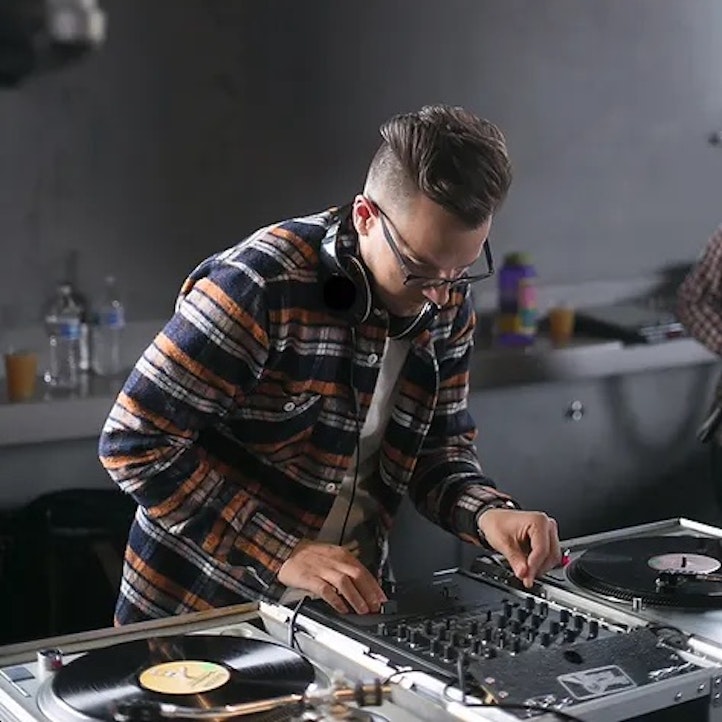This color photograph, presented in a square format, captures a detailed scene of a young male DJ, approximately 30 years old, deeply engrossed in his work. Standing at a mixing table, he manipulates a sound mixer board flanked by two turntables, each holding a vinyl record. His attire includes a Pendleton-style plaid shirt with hues of blue, orange, and white, worn open over a white t-shirt. He accessorizes his look with dark glasses and a pair of headphones resting around his neck. The DJ's hair is short and shaved on the sides, poofed up on top, and he gazes downward towards the right side of the image, focusing on his craft.

The background features a gray, possibly metal or ceramic, setting that includes countertops slightly out of focus. Atop these surfaces, there are small but distinct details such as bottles of mineral water to the left of the frame, a hint of soap or another item to the right, and an unlit light fixture. The scene embodies a realistic photographic style, emphasizing the professional yet intimate environment of the DJ at work.